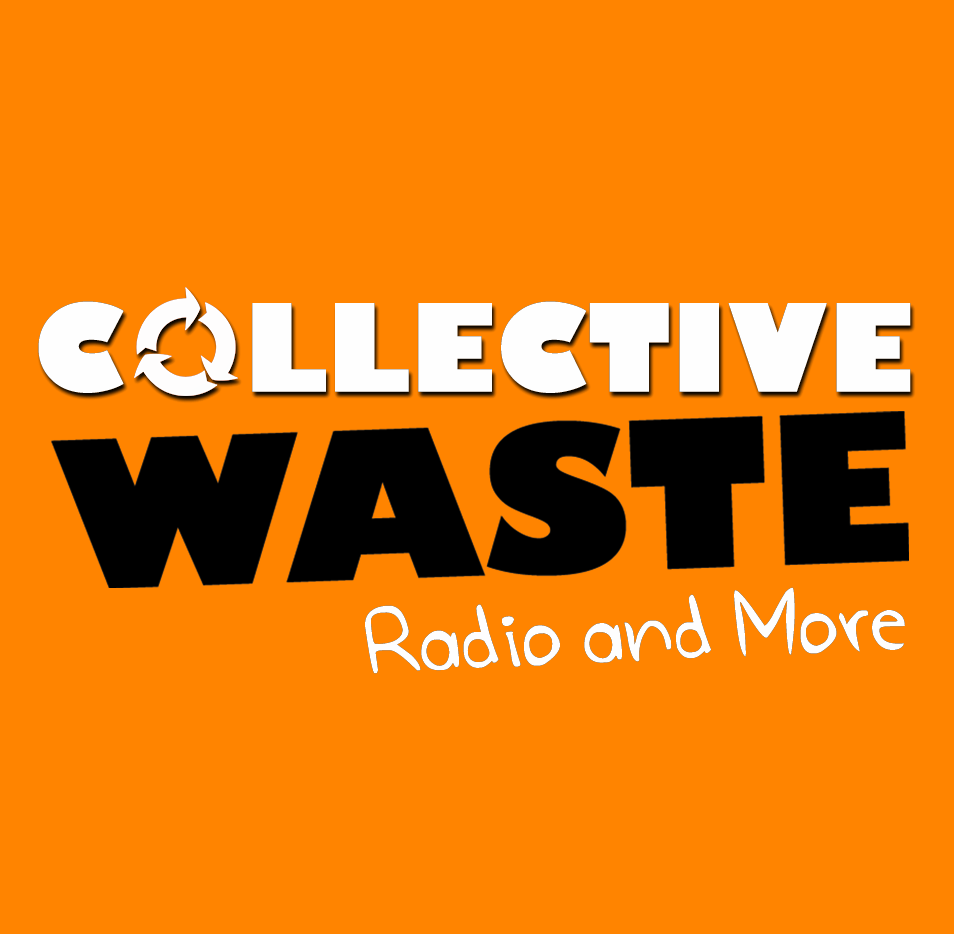The image features a solid orange background with centered, stylized text. At the top, the word "Collective" is displayed in thick, white uppercase font, with the "O" replaced by a recycling symbol composed of three arrows forming a circle. Below it, the word "Waste" appears in large, bold black font, slightly angled. At the bottom, "Radio-N-Moore" is written in a thin, chalky white font that mimics handwriting. The composition appears to be a title or cover image, potentially for a podcast or blog focused on recycling and waste management. Its distinctive fonts and recycling motif suggest it could be used for a website or promotional materials in residential areas to educate and inform the public on environmental practices.